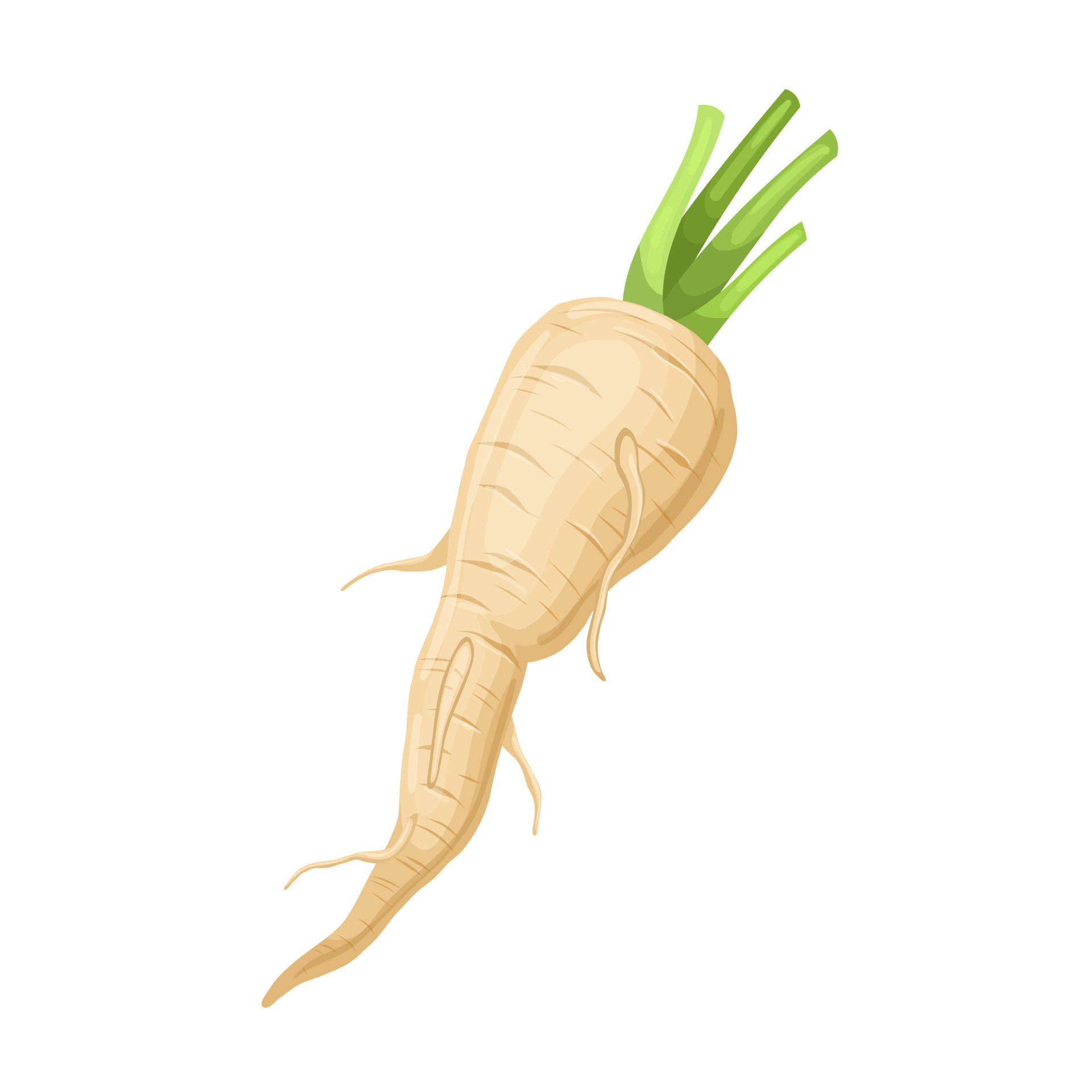This image is a detailed cartoon drawing of a root vegetable, most likely a radish, depicted on a pure white background. The vegetable is light brown to tan in color and is shaped like a tapered root, starting wide at the top near the soil and narrowing to a point at the bottom. It is oriented diagonally from the bottom left to the top right. Several small offshoots and thin, cylinder-like protrusions extend from the root, and dark brown dash lines are scattered across its surface. Four green stems emerge from the top of the radish, with two stems being darker green and the other two lighter green. These stems are depicted as wavy, vertical rectangles, adding a touch of organic texture to the drawing.